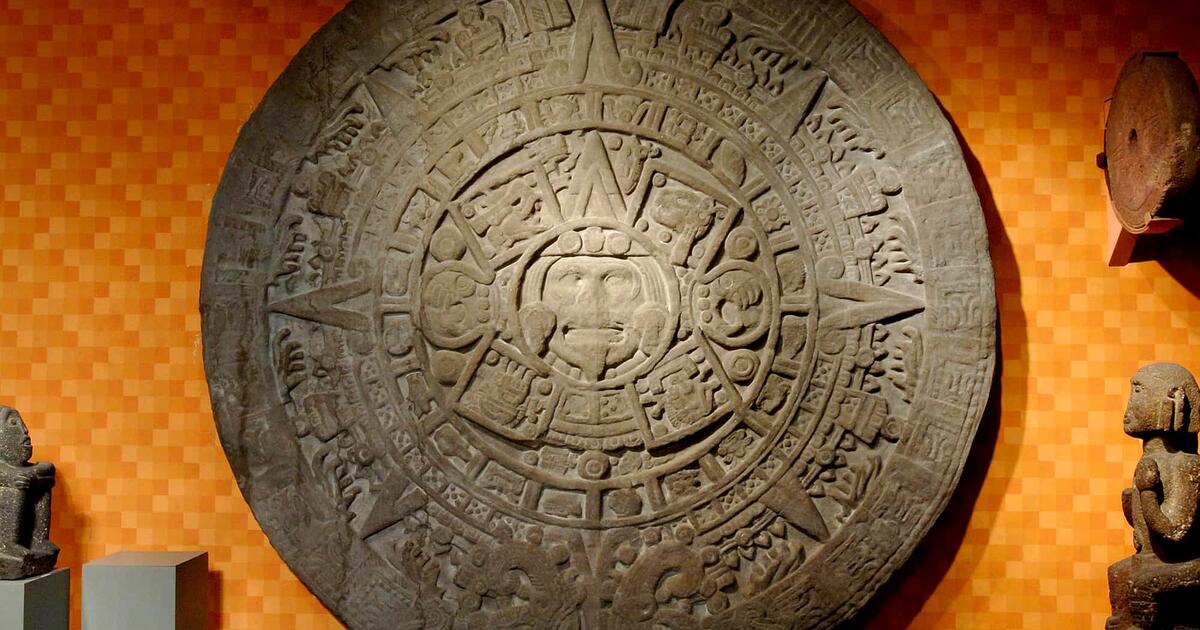This photograph vividly captures an ancient artifact reminiscent of Mayan architecture, specifically invoking the appearance of an Incan sundial wheel. The central object is a large, grayish, pewter-colored stone disk adorned with intricate geometric designs, including squares and triangles, reminiscent of Mayan civilization and featuring Roman numerals. At its core, there is a relief or carving of a human face with distinctive features such as eyes, a mouth, and potentially a goatee, giving it a regal presence. This artifact is set against a striking orange checkered background, composed of varying shades of light and dark orange. Surrounding the main disk are several pedestals and smaller artifacts, including statues observing the disk. The entire scene emphasizes the ornate detail and historical significance of the central artifact, making it a visually compelling and detailed representation of ancient craftsmanship.